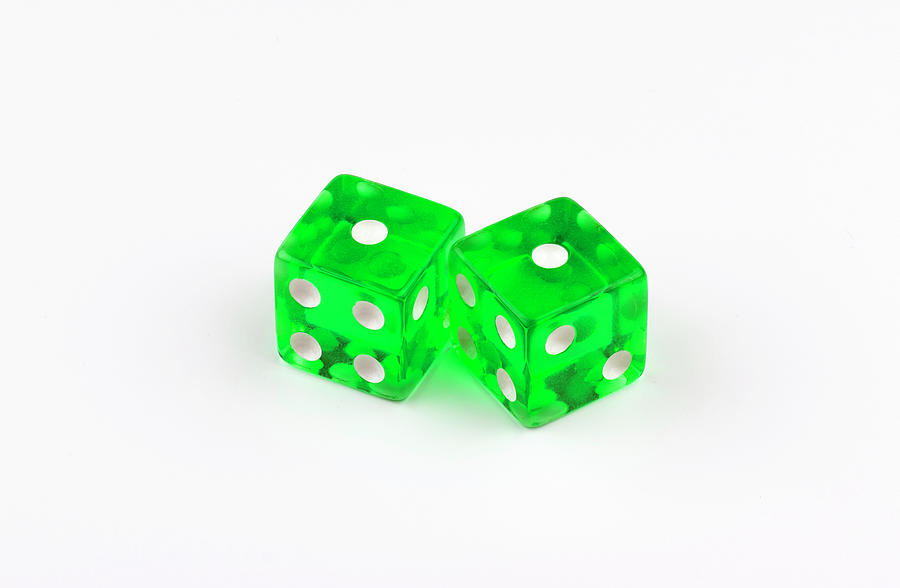This image features a visually striking pair of green fluorescent dice with white dots, positioned centrally on a stark white surface. The dice display the number one on the top face of each, symbolizing snake eyes. The left die shows the number four on its forward-facing side, while the right die, positioned at a slight diagonal, reveals the number four on its left and the number two on its right. The minimalist background accentuates the vivid green hue and the partial transparency of the dice, emphasizing their stark contrast against the white backdrop.